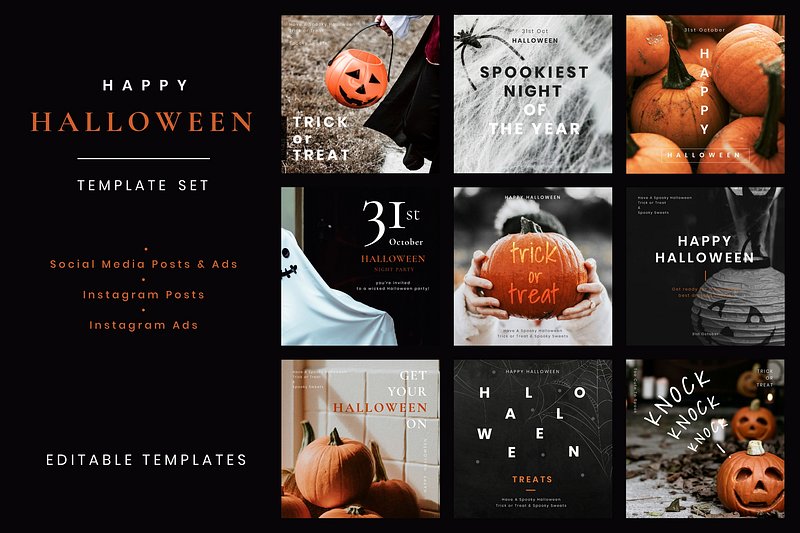This image appears to be a part of a website or an app, specifically a section showcasing a set of customizable templates for Halloween-themed social media posts and advertisements. The section title on the left reads "Happy Halloween Template Set," emphasizing that these templates are editable for use on platforms like Instagram.

Nine distinct templates are displayed on the right:

1. **Trick or Treat**: Features an image of a child's hand and leg, dressed possibly in a vampire outfit or a black dress, holding a plastic pumpkin with a jack-o'-lantern face for collecting candy.
2. **Spookiest Night of the Year**: Showcases a spider sitting in the center of an intricate spider web.
3. **Happy Halloween**: Displays an array of uncarved pumpkins.
4. **31st October Halloween**: Centers around a graphic of a smiling ghost reminiscent of a sheet draped over an object, with expressive eyes and a mouth.
5. **Trick or Treat**: Depicts a person holding a pumpkin up towards the camera, highlighting the festive spirit.
6. **Happy Halloween**: Shows an IKEA-style paper lantern lamp with a jack-o'-lantern face, adding a decorative touch.
7. **Get Your Halloween On**: Features a photograph of several uncarved pumpkins lined up along a tiled wall, similar to a kitchen setting.
8. **Halloween**: The word "Halloween" is written with letters placed at varying heights, creating a playful and distorted effect.
9. **Knock Knock**: Presents a trio of carved jack-o'-lanterns, each with distinct, cute facial expressions.

These visual elements collectively provide a diverse range of options for engaging and festive Halloween content.